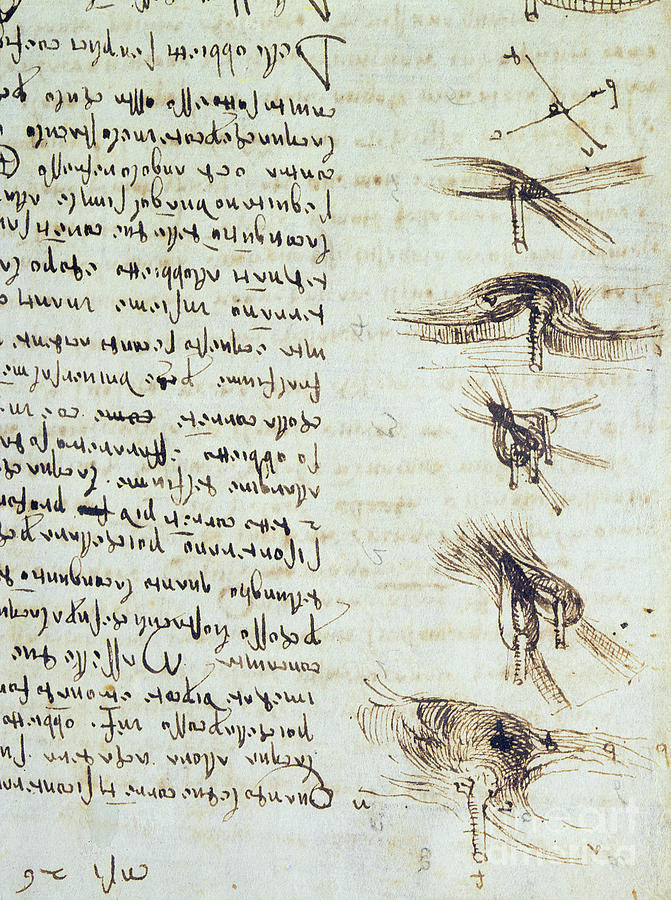The image depicts an old piece of parchment, possibly Manila, showcasing intricate scientific diagrams and illustrations by Leonardo da Vinci, known as the Codex Leicester. On the right side of the page, five detailed pen and ink drawings are visible, with one featuring an X at the top adorned with smaller symbols at each end. These sketches, which include looping structures resembling hair and pillars, are part of da Vinci's extensive work on anatomy and science. The left side of the page contains several lines of text in a foreign language, written in da Vinci's characteristic reversed script, suggesting it should be read from right to left. The black ink text is so finely executed that it bleeds through the parchment, making the writing on the back partially visible.